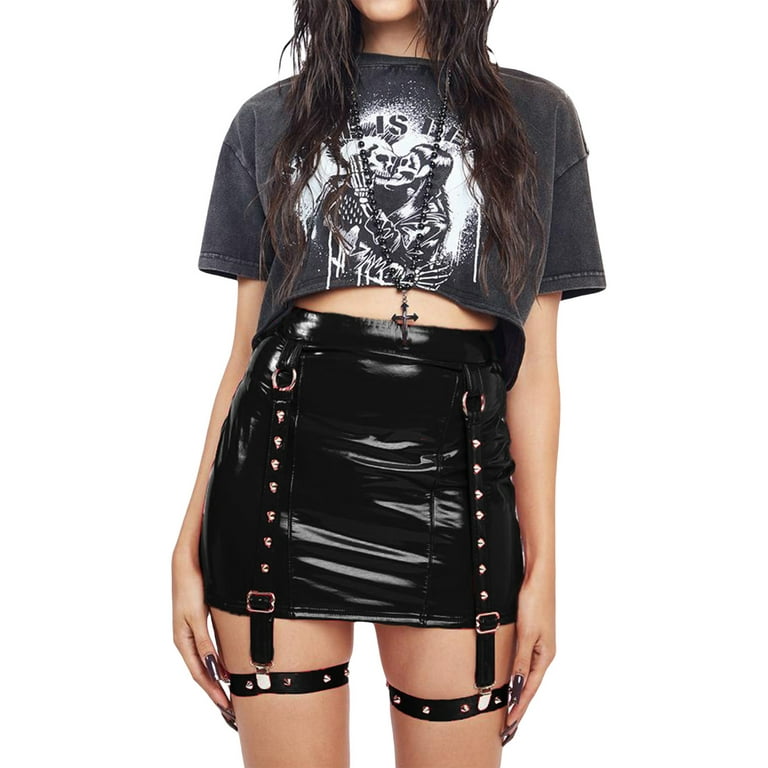In this color photograph set against a white background, a young female model with long, dark brown hair is depicted from the chin down to just above her knees, with her face not visible. She is modeling a black crop top t-shirt featuring a black and white image of a male and female skeleton, with the male skeleton having a mohawk. The skeletons are depicted in an intimate embrace. The model is also adorned with a long black rosary necklace that extends down to her midriff and wears a tight, black patent leather mini-skirt that is very short. The skirt has thigh straps attached with gold buttons that wrap around her thighs, and there are chains hanging down from both sides of the skirt. Her arms rest at her sides, with her hands on her thighs, displaying black nail polish.